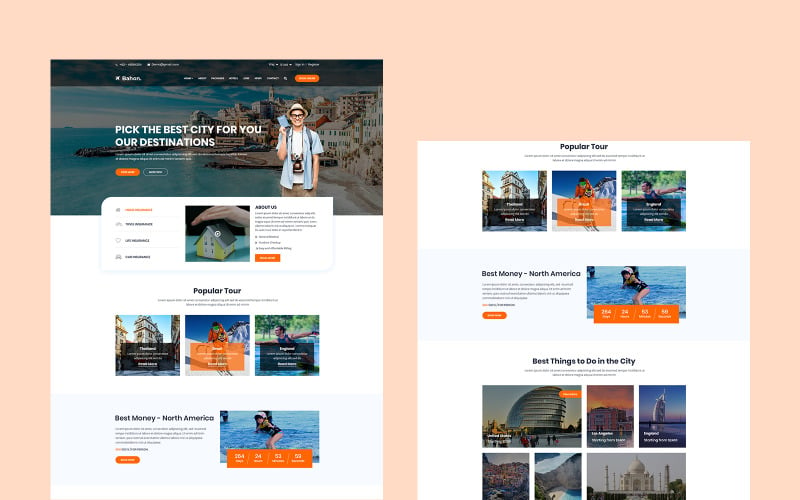The image features a vibrant pink background with a central page depicting a picturesque coastal village or city by the sea. The scene captures a serene beach, historic-looking buildings, and a tranquil ocean meeting a clear blue sky. A character resembling a tourist stands prominently, dressed in a short-sleeved blue shirt, a wide-brim hat, and a camera slung around their neck. They hold a book, apparently a travel guide. Above this engaging scene, there's text saying, "Pick the best city for you, our destinations." Below this phrase is an unreadable sentence, followed by two buttons: one orange and the other mirroring the water's hue in the image.

Beneath this main section is a smaller photo of a miniature house with a person's hand hovering above it. The words "Popular Tour" accompany this image. Below the "Popular Tour" label are three thumbnails: the first shows a building, the second depicts a skier on a mountain slope, and the third appears to show someone swimming, though it's not entirely clear. Another text statement reads, "Best Money North America."